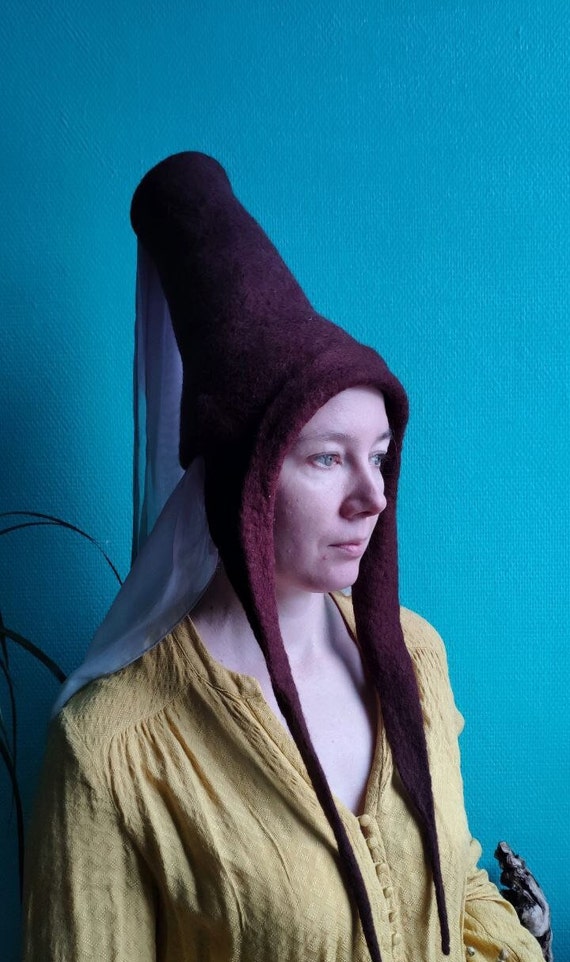A portrait of a modern-day, Caucasian woman is depicted wearing Renaissance-style clothing. She gazes contemplatively to the right, her face framed by a tall, narrow, dark maroon hat made of wool or felt, adorned with a silk veil cascading from the back and two long strips hanging down to her chest. Her blue eyes and middle-aged facial features, including a prominent nose and pink lips, are accentuated by her light skin tone. She is dressed in a mustard-colored, long-sleeved, button-up shirt with a v-neck, the fabric of which is cotton. The background is a bright blue-green turquoise, and her upper body is framed by a large plant whose limbs reach shoulder height. The bright setting and historical attire create a striking contrast, with the woman appearing lost in thought, yet poised and composed.